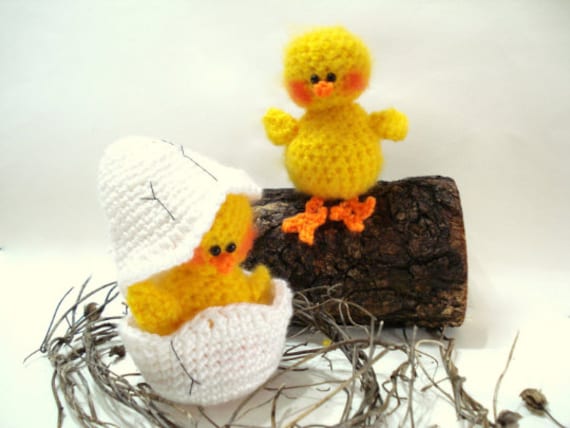The image displays a detailed crocheted scene on a light gray background, presented in a landscape orientation. Central to the composition is a yellow crocheted chick with black bead eyes, a small orange beak, pink-orange cheeks, and matching orange feet. The chick is positioned confidently on a horizontally placed brown log, approximately six inches wide and four inches deep. Surrounding the log is a circular arrangement of small twigs forming a nest-like structure.

To the bottom left of the log, nestled within the twig circle, sits a white crocheted egg, cracked open to reveal another baby chick inside. This secondary chick, crafted similarly to the one on the log, peeks out from the partially open egg shell, which features a zigzag edge with black accent stitching.

The entire scene, highlighted by detailed crocheted elements and accent stitching, captures a charming and whimsical representation of two baby chicks, one prominently displayed on the log and the other emerging from its egg, all set against a minimalist backdrop.